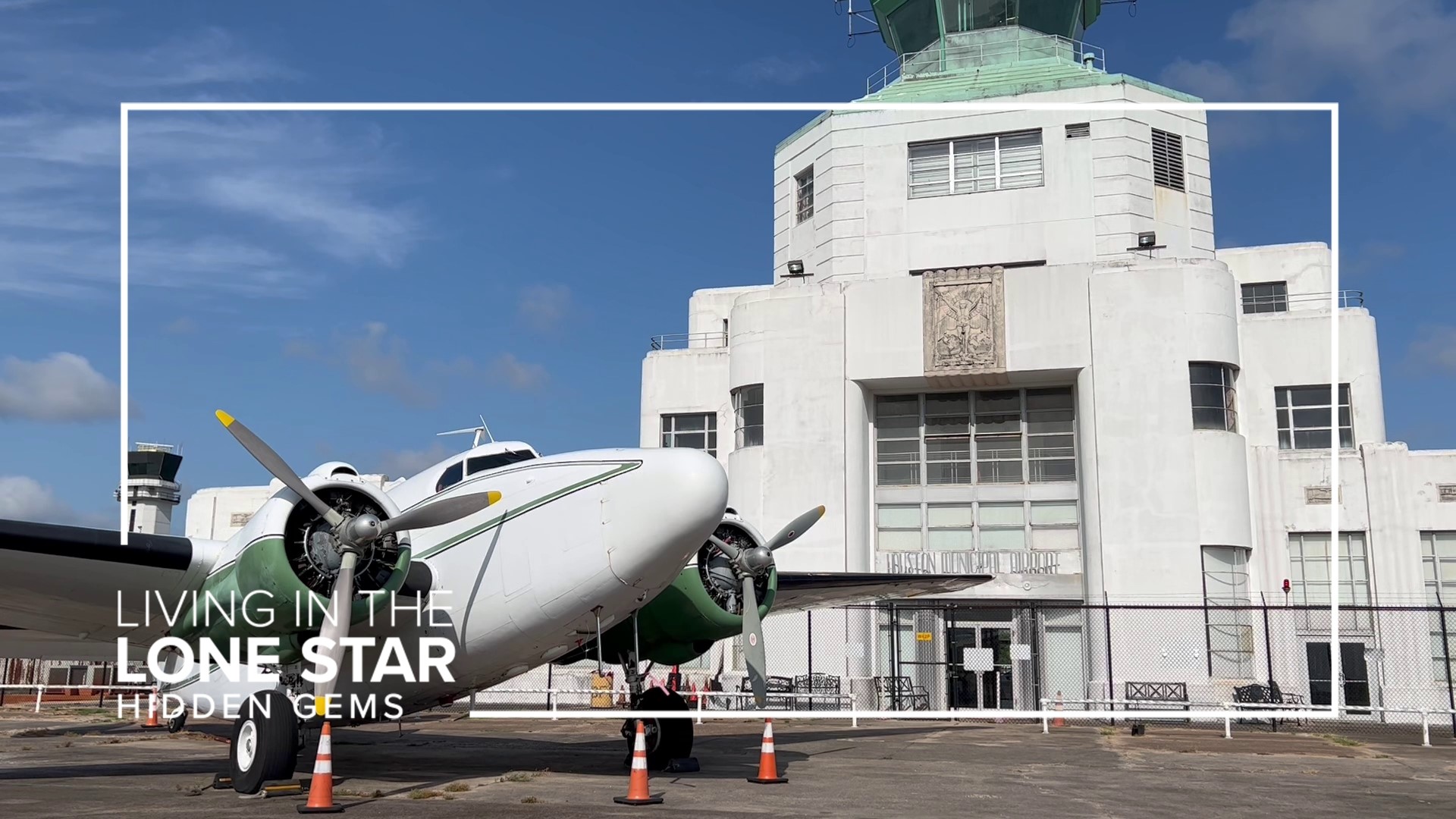A captivating image reminiscent of a tourist brochure showcases the Houston Municipal Airport, with a prominently featured white propeller plane in the foreground. This plane, distinct with its dual green-painted engines on each wing, hints at the adventurous spirit of independent aviation. Dominating the background is a cream and brown building, atop which stands a control tower, essential for overseeing the airport's activities. The building also proudly displays an emblem. Set against a sky dotted with clouds, the image is accentuated by unreadable text, with a highlighted rectangle at the bottom left stating, "Living in the Lone Star Hidden Gems," adding to the allure of this Texas treasure.